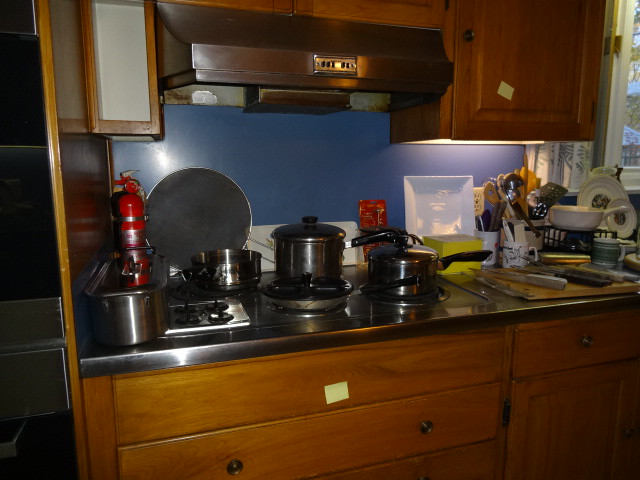A cozy, albeit cluttered kitchen scene is depicted in this photograph. The focal point is a stovetop adorned with three pots and a frying pan, all actively in use, suggesting a bustling cooking session. Above the stove, a ventilator system integrated into the bottom of a microwave hints at functionality, designed to whisk away steam and smoke. The kitchen features an older aesthetic, characterized by dark brown cabinets, lending a rustic charm. Two yellow sticky notes provide bursts of color and hint at reminders or instructions; one is affixed to an upper cabinet door and another to a drawer below the stove. A stainless steel container and a fire extinguisher occupy the back corner of the stove area, reinforcing both convenience and safety. 

A blue wall backdrop contrasts pleasantly with the kitchen's warm wood tones. Leaning against the wall, a strainer awaits its next use. To the right, the countertop is a symphony of culinary tools and ingredients—dishes are scattered haphazardly, and a cutting board, complete with laying knives, points to ongoing meal preparation. Open containers overflow with spatulas and wooden utensils, ready to play their part in the cooking process. The scene is completed with various plates and bowls, exemplifying the organized chaos of an engaged home cook.